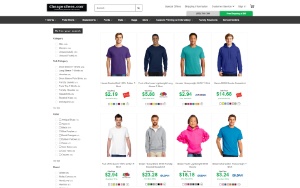Here is a cleaned-up and detailed caption for the image:

This image is a slightly blurred screenshot of an e-commerce website specializing in men's clothing, even when zoomed in. The website's interface includes a search bar positioned above the header, along with two adjacent tabs located on the upper-right corner; the left tab is gray while the right tab is green. The website predominantly showcases apparel suitable for summer and spring. 

The top row features male models displaying various outfits, and the bottom row also includes male models except for the third image from the left, which depicts a young boy wearing a pink hoodie. The price range of the garments spans from approximately $2 to $35. The least expensive item is a teal shirt priced at $2.94, appearing as the third item from the left in the top row. Conversely, the priciest item is a gray hoodie, modeled by the second person in the second row, costing $33.38.

Additionally, the right side of the website features a section allowing users to filter clothes based on criteria such as sex, size, style, and brand.